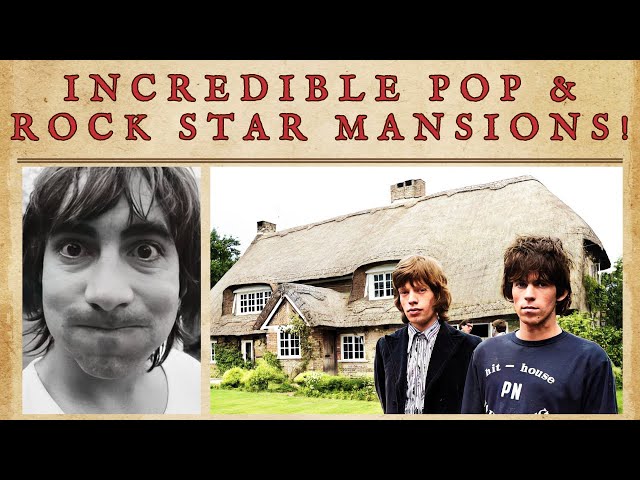This image is a detailed poster featuring young Mick Jagger and a fellow band member, both standing in front of a quaint English cottage. Mick Jagger is dressed in a black, velvety-looking suit jacket with a striped collared shirt, while the other man wears a blue sweatshirt. Both men have long, shaggy brown hair. The quaint stone house with a gray roof is set behind them amidst lush green grass and bushes, under a white cloudy sky. There is a black-and-white close-up photo of a man on the left side of the poster, with tousled brown hair, thick eyebrows, wide eyes, and puffed-up cheeks, as if he's holding his breath. The entire image is framed with black borders at the top and bottom, and a brown border that displays the red block text: "Incredible Pop and Rockstar Mansions!"